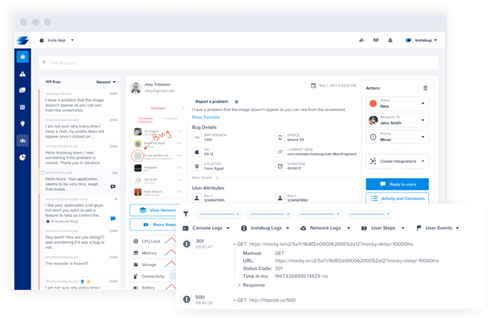The image displays a screenshot of a website interface. At the top of the page, there's a light gray navigation bar. On the upper left corner of this bar, three gray circles are aligned horizontally. Below the gray bar, there's a white bar containing a logo comprised of dark blue and neon blue squares. To the right of the logo, there is a tab, while in the upper right corner of the page, we can see several icons, including one that resembles a notification bell.

The left side of the page features a vertical strip of seven white icons. Dominating the center section of the image is a large amount of text interspersed with various icons and buttons. Notably, there is an element highlighted with a red circle, accompanied by a red arrow pointing towards it with the label "bug." The image quality is quite poor, making it difficult to discern finer details clearly.